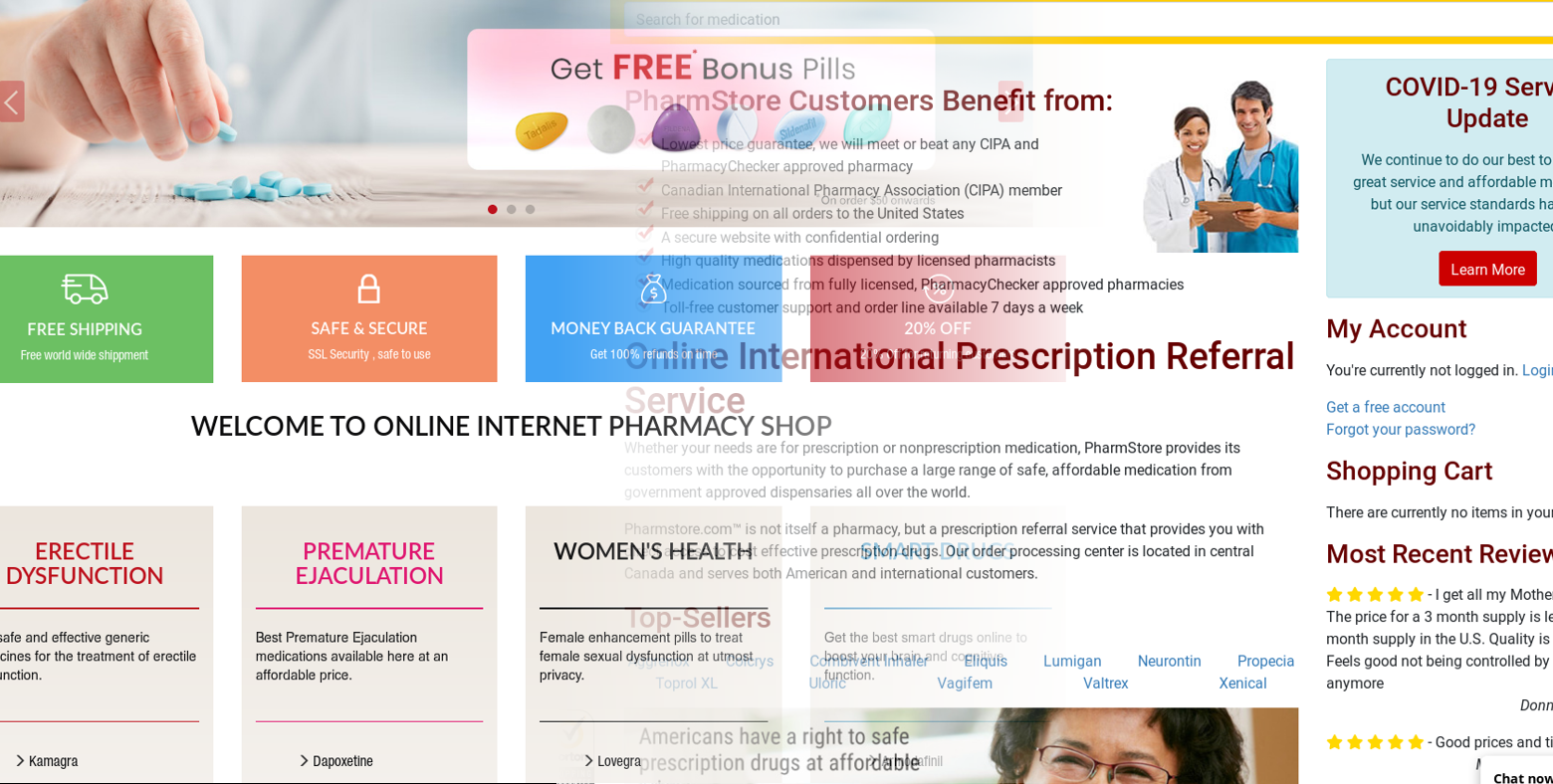This image captures a vibrant website, likely viewed on a computer. The website features a predominantly white backdrop, accentuated by a series of colorful squares at the top. Each square highlights a different service aspect: the green box indicates free shipping, the orange signifies a safe and secure site, the blue promotes a money-back guarantee, and the red offers a 20% discount. Centrally located on the page is a black-lettered welcome message that reads, "Welcome to Online Internet Pharmacy Shop." The site also includes a red-lettered shopping cart icon on the right-hand side. Toward the bottom of the visible section, there's a section labeled "Most Recent Review," showcasing a five-star rating for the site. The overall design is both functional and visually appealing, with the colorful elements drawing attention to key features and benefits for potential customers.